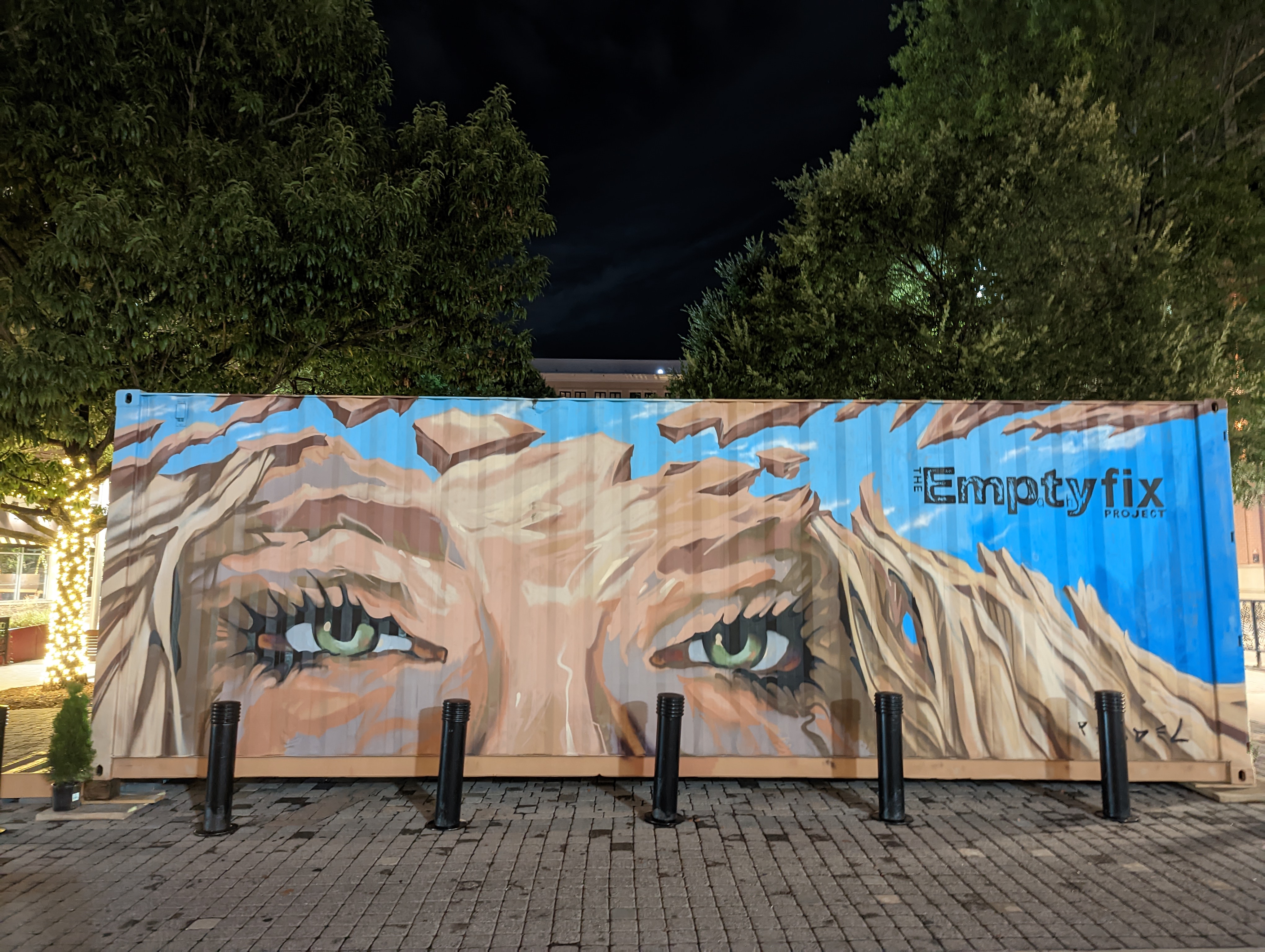In a dimly lit park or city square at night, the focus of the image is a giant shipping container adorned with a striking mural. The artwork, which spans about 20 feet in width and 5 to 6 feet in height, prominently features the face of a woman from the nose up, with an emphasis on her piercing green eyes and flowing blonde hair, depicted in an almost wood-like texture. The mural is set against a background of sky blue, and in the upper right-hand corner, it reads "The Empty Fix Project" in black ink. Surrounding the container, the area is paved with brick, and in the background, the tops of two large trees are visible, adorned with lights that add a subtle illumination to the scene. In front of the mural, there are also five black pillars, adding to the urban ambiance.